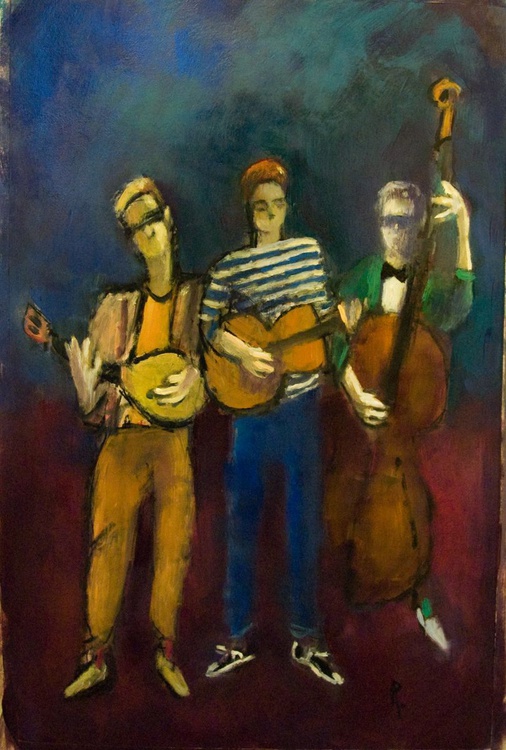The image is an impressionistic color painting in portrait orientation, depicting a three-member band ensemble. The figures are positioned close together against a vibrant backdrop, with the top half featuring bright blue and dark teal brushstrokes, and the bottom half highlighted by dark red and black strokes. 

The musician on the left is a blonde man wearing sunglasses and beige trousers. He is playing a ukulele or mandolin-like instrument, though it appears slightly distorted in design. The central figure is a young man with reddish-brown hair, dressed in a blue and white striped shirt and blue jeans, playing a clear classical guitar. To the right stands a man in a green tuxedo jacket, complete with a black bowtie and a white shirt. He has light beige hair and is playing a large cello that rests on the floor. Notably, the figures lack mouths and have minimal facial details, emphasizing the impressionistic style of the artwork.